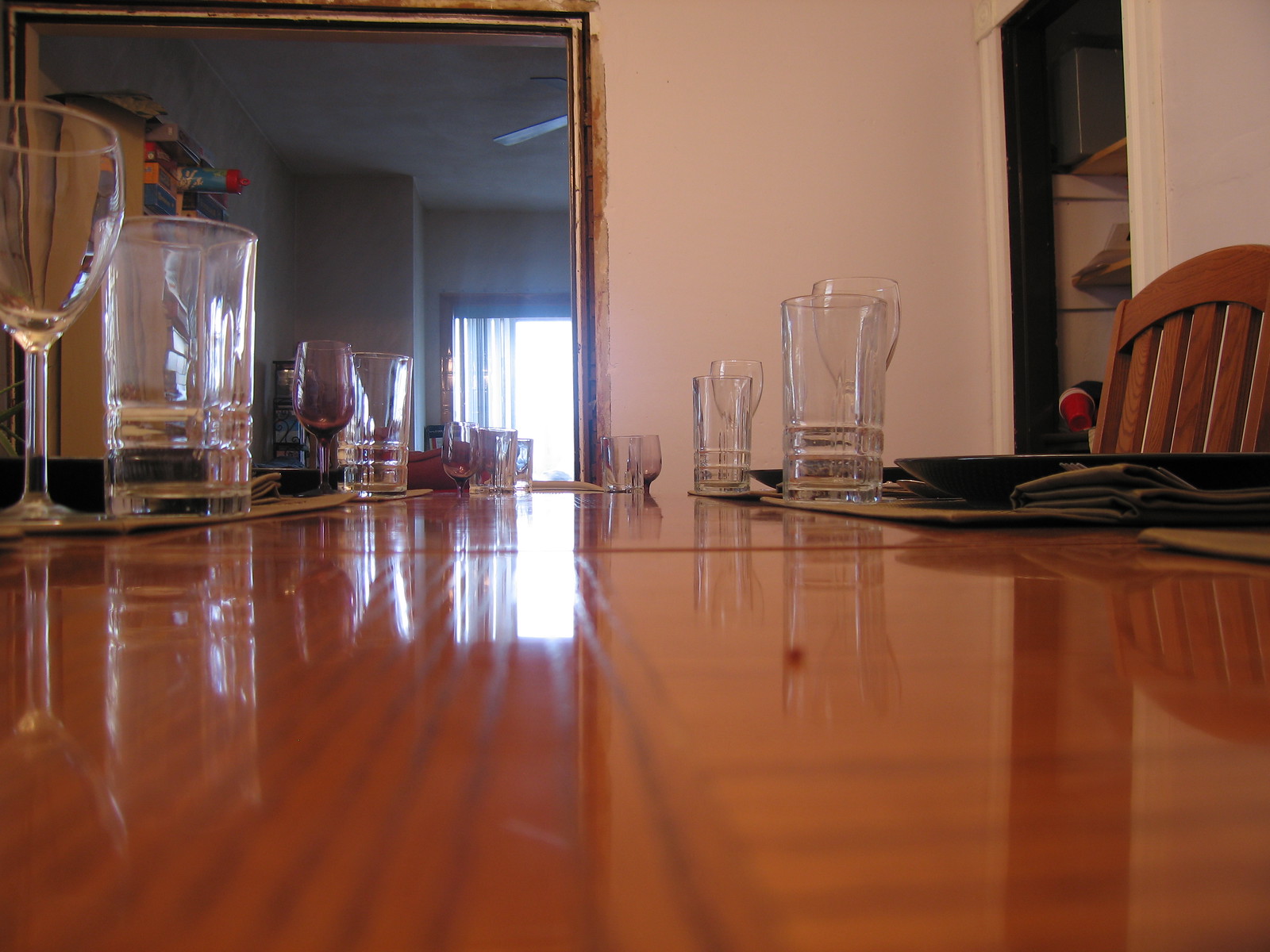This photograph captures an elegant dining room set for a meal, viewed from the perspective of someone seated at the table. The table itself is crafted from wood and features a highly reflective, glossy finish that adds a touch of sophistication to the scene. Adorning the table are clear water and wine glasses, meticulously arranged, along with neatly placed plates and napkins, suggesting that the meal is about to begin. A wooden chair is partially visible, indicating a comfortable seating arrangement. The room is characterized by pristine white walls and glossy white trim, which contribute to the clean and inviting atmosphere. The dining area opens into an adjacent room through a double-case opening, where a window allows natural light to stream in, enhancing the overall warmth and brightness of the space. The meticulous table setting and the serene ambiance promise an enjoyable upcoming meal in this charming dining room.